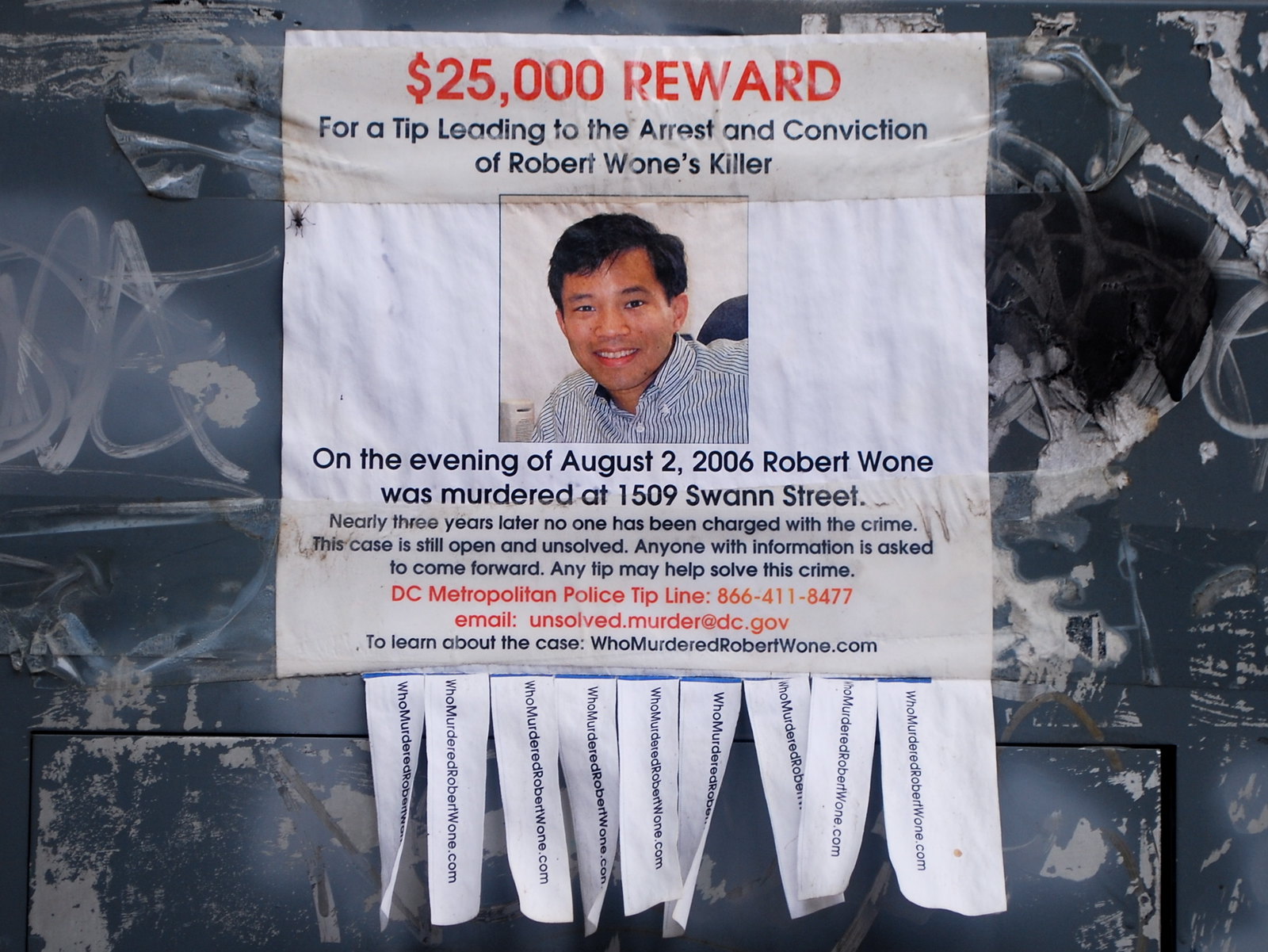This image shows a flyer pinned to a metal structure, detailing a $25,000 reward for information leading to the arrest and conviction of Robert Wone's killer. The flyer, taped securely, features the smiling face of Robert Wone, a young man with short dark hair, wearing a white shirt with blue stripes. Bold red text at the top announces the reward amount. Below his picture, the flyer states that on the evening of August 2, 2006, Robert Wone was murdered at 1509 Swan Street. Nearly three years later, the case remains open and unsolved. It urges anyone with information to come forward, as any tip could help solve the crime. The flyer provides contact details for the DC Metropolitan Police tip line at 866-411-8477 and an email address at unsolved.murder@dc.gov. Additionally, there is a URL for more information on the case at whomurderedrobertwone.com. At the bottom of the flyer, small tear-off strips are available, each printed with the same web address.